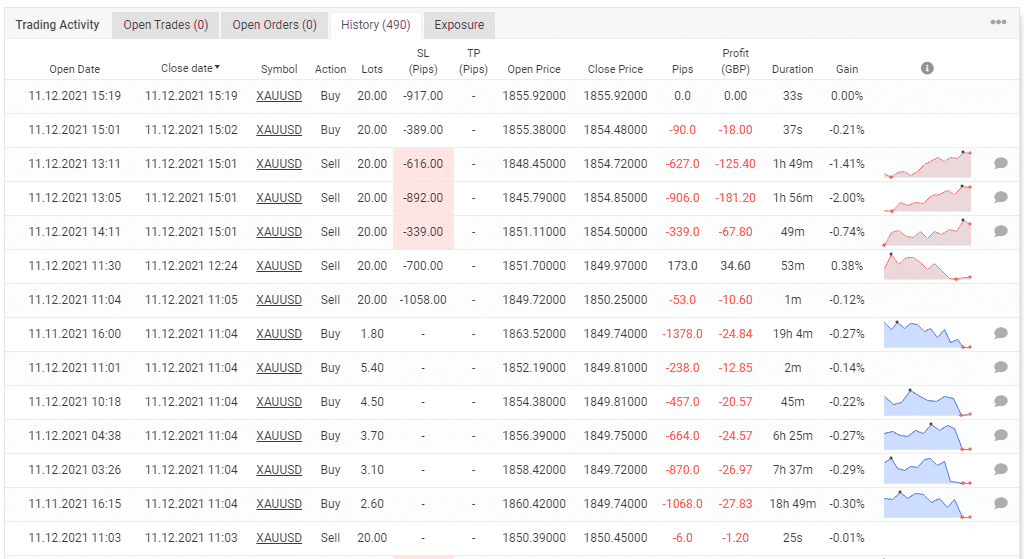The image is a screen capture from a trading application or website, showcasing trading activity under the 'History' tab. The top left corner features a series of navigational tabs labeled: 'Trading Activity', 'Open Trades', 'Open Orders', 'History', and 'Exposure', with the 'History' tab currently highlighted. In the upper right-hand corner, there's an icon with three dots, indicating a drop-down menu is available.

The main section of the image is organized into a table format, consisting of rows and columns, each with distinct headings. The columns are as follows:
- **Open Date**: Lists the dates when trades were opened.
- **Closed Date**: Displays the dates when trades were closed.
- **Symbol**: Shows the trading symbol, 'XAUUSD', which appears to be consistent across all entries and likely represents a gold (XAU) to U.S. Dollar (USD) currency pair.
- **Action**: Indicates the type of trade, either 'Buy' or 'Sell'.
- **Lots**: Ranges from 1.8 to 20, depending on the individual trade.
- **SL Pips**: Displays 'Stop Loss' pips for the first seven trades, with the rest left blank.
- **TP Pips**: Is blank for all trades, indicating no 'Take Profit' pips were set.
- **Open Price**: Lists the price at which each trade was opened.
- **Closed Price**: Shows the price at which each trade was closed.
- **Pips**: Reveals the gain or loss in pips, either positive or negative.
- **Profit**: Shows the monetary profit or loss, denoted as positive or negative values.
- **Duration**: Indicates how long each trade was open.
- **Gain**: Details the overall gain for each trade.

The detailed breakdown of the columns provides a comprehensive view of the trader's historical activity, reflecting both profitable and loss-making trades in terms of pips and monetary values.